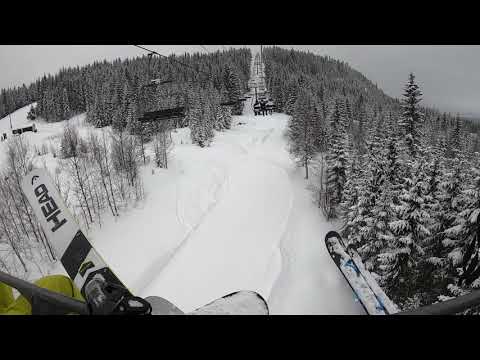In this dynamic black and white image, we observe skiers from an overhead perspective as they ride a ski lift up a snowy mountain. The scene is dominated by an expanse of white snow, creating a stark contrast with the dark, densely packed pine trees whose branches are laden with snow. The snow-covered trees are concentrated on the lower right-hand side while smaller snow-dusted trees pepper the right-hand side of the image. 

The photograph appears to have been taken with a GoPro, giving it a slight fisheye effect. In the lower left and right-hand corners, the skis and lower legs of the skiers come into view. One skier is dressed in spearmint green snow pants, while their companion sports yellow pants. The skis in the frame are distinct; one is white with a black stripe and the brand “HEAD” visible in black text, while another ski, belonging to the person on the right, appears to be black and blue.

A horizontal wire holding empty ski lift chairs stretches diagonally across the scene, reinforcing the motion and ascent up a white, meandering trail that snakes toward the mountain's peak. Dark horizontal black strips frame the top and bottom edges of the image, centering attention on the serene yet exhilarating winter landscape and the skiers’ journey up.